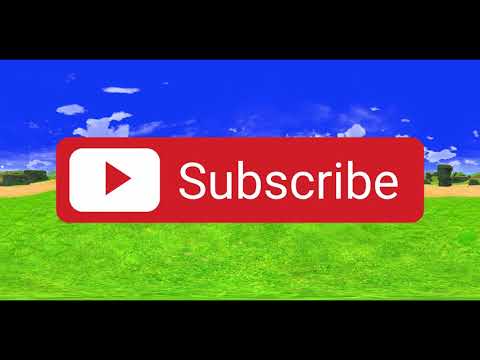The image prominently features a red YouTube "Subscribe" button set against a backdrop of a Minecraft scene, characterized by vivid green grass, a deep royal blue sky, and a few low-lying white clouds. A strip of sand is visible before a line of pixelated trees. The scene is slightly less rendered than typical, adding to the pixelated aesthetic of Minecraft. The YouTube button is shown as a white square with a red rectangle in the center and white text. The image has black bars at the top and bottom, mimicking the appearance of a YouTube video frame.